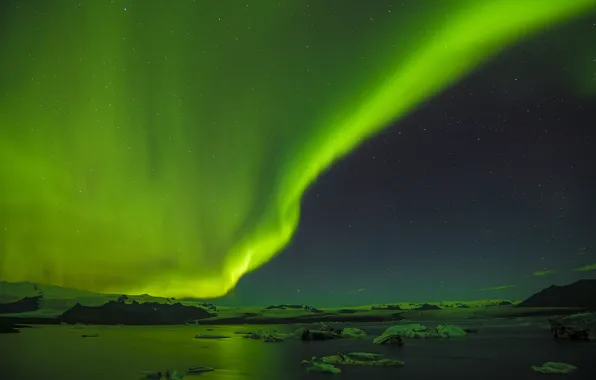The night setting captures a breathtaking arctic landscape, characterized by a serene body of water peppered with small icebergs. The sky is dramatically split, with a luminous green aurora dominating the left side, blending into shades of blue, green, and purple as it extends toward the center. Tiny clouds linger in the distant background, and a sprinkle of stars is visible across the top part of the image. On the right, the dark sky contrasts sharply with the aurora's brilliance, revealing a bit of land with gentle slopes, possibly walked upon, in the horizon. This enchanting scene exudes the chilly calm of a cold environment, enhanced by the captivating natural light show of the aurora borealis.